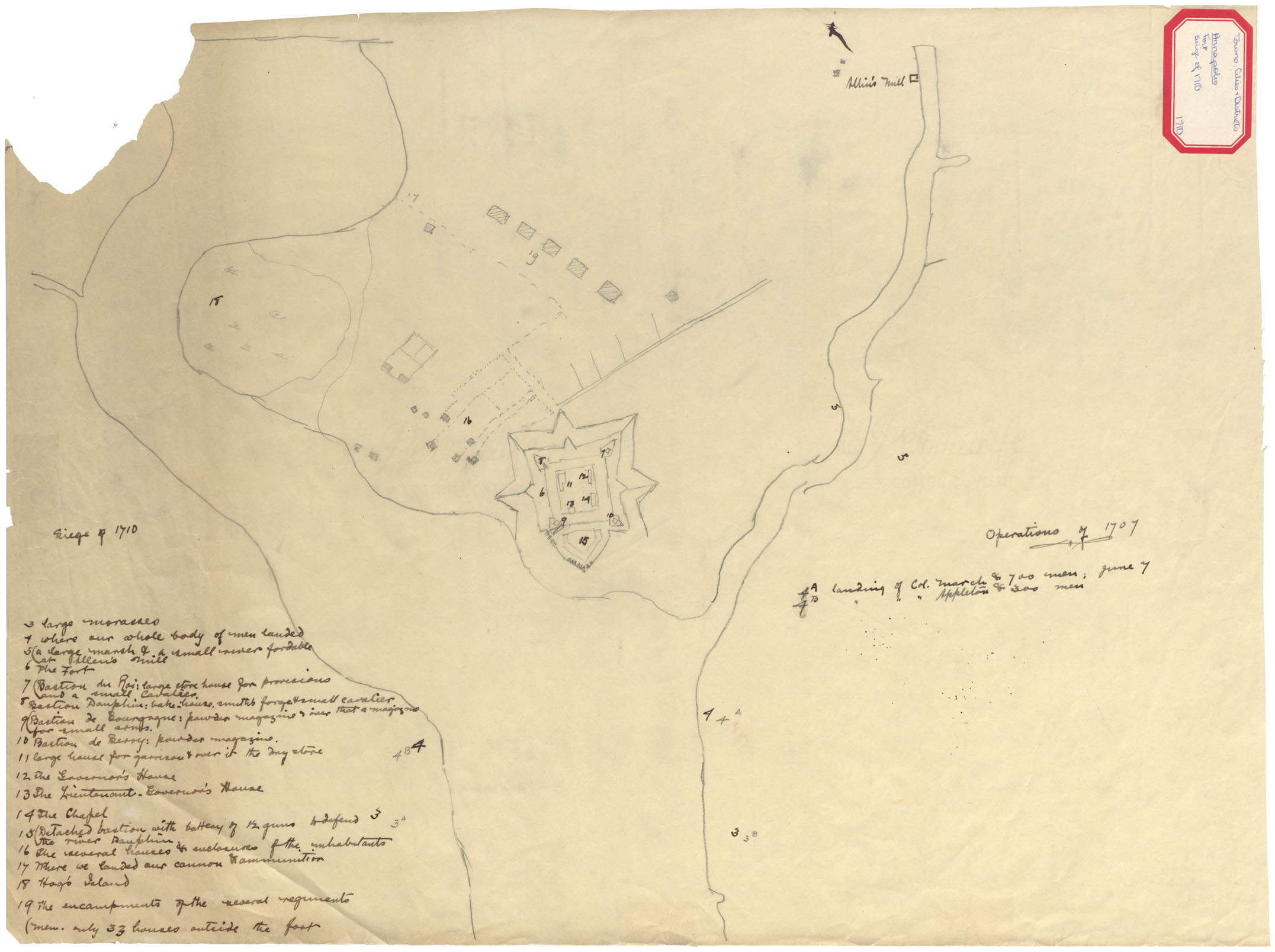The image captures a hand-drawn map on an aged, sepia-toned paper, torn at the top left corner. The map features intricate details such as roads or rivers, and blueprints of various areas, with significant handwritten annotations. In the middle of the map, there is a star-shaped courtyard, central to the layout, with additional smaller images and markings around it. A building with a four-pointed edge and a square center is prominently drawn, surrounded by what resemble trails branching out, a parking lot area with lined spaces, and a possible tennis court and pool or pond. On the left side, rows of numbered handwritten notes reference places on the map, including 'Siege of 1710,' although the writing is difficult to decipher. In the top right corner, a red vertical hexagonal box contains notes mentioning 'Town of Celesie,' 'Tuesday Trust,' 'Amno Polio Fort,' and 'Siege of 1710,' providing context to some of the map's features. The paper is crinkled and smudged, emphasizing its age and the wear it has endured over time.